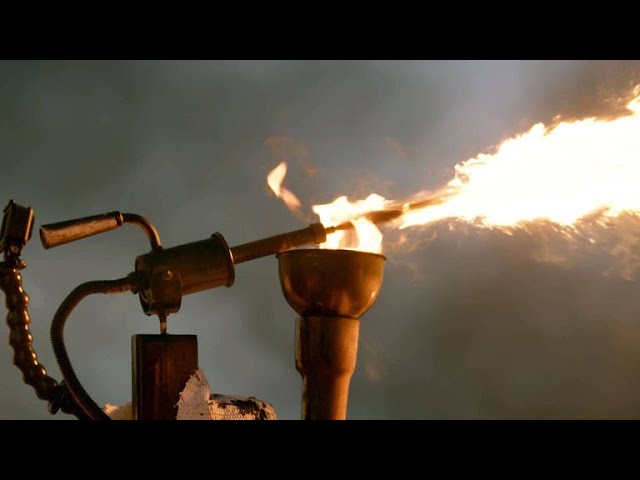This color photograph captures a close-up view of a brass torch being used to heat metal. The image is bordered by black at the top and bottom, while the central background displays a grayish, cloudy color. A prominent orange flame flares out to the right, emitted from a metal nozzle which is intricately designed with a wavy structure at the back. This nozzle is likely shooting out a flammable liquid that ignites to create the intense fire. The torch features a black handle with a turn crank and seems to be connected to a copper pipe. Despite the dark gray and light gray hues in the background, the entire scene is brightly illuminated, possibly from the intense flames or additional lighting. Smoke surrounds the area, further suggesting high heat and combustion. This could be a snapshot from a movie or a YouTube video demonstrating the operation of a flamethrower-like device.